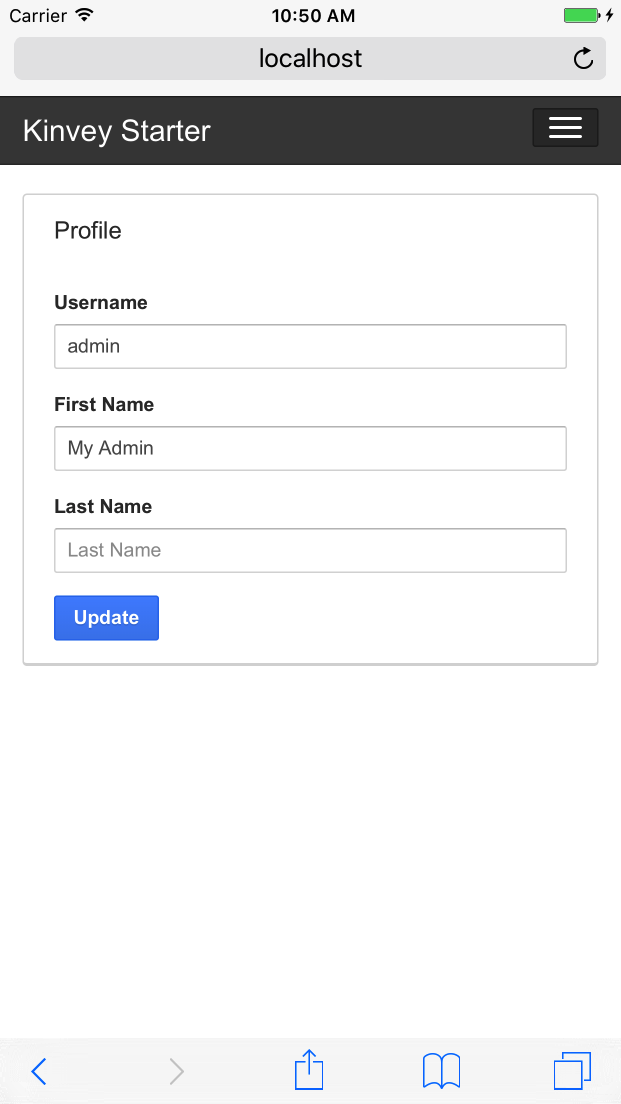The image depicts a screen grab from a smartphone, showcasing an app interface. The frame is vertically rectangular, with various icons and text arranged neatly across the screen. 

At the very top of the screen, on the left-hand side, the word "Carrier" is displayed, accompanied by a Wi-Fi icon to its right. Centrally positioned is the time, "10:50 AM," while the battery icon appears at the top right corner.

Just below the time, the text "Local Host" can be seen. Directly beneath this, on the left, it says "Kinbee Starter," accompanied by a menu bars icon on the right. Both of these elements are placed under a solid black horizontal banner.

Moving downwards, there is a gray outlined square taking up a significant portion of the screen. Within this square, the content is left-aligned and begins with the word "Profile." Immediately below, there’s an input field labeled "Username," which currently displays the text "admin." 

Following that is another input field labeled "First Name," containing the text "My Admin." Subsequent to this is a field labeled "Last Name," which is currently empty, displaying the placeholder text "Last Name" in gray.

A blue button with the text "Update" in white letters is located beneath these fields.

At the very bottom of the frame, there is a navigation bar that includes a blue back arrow, a gray forward arrow, an upload icon, a book icon, and a copy icon, from left to right.